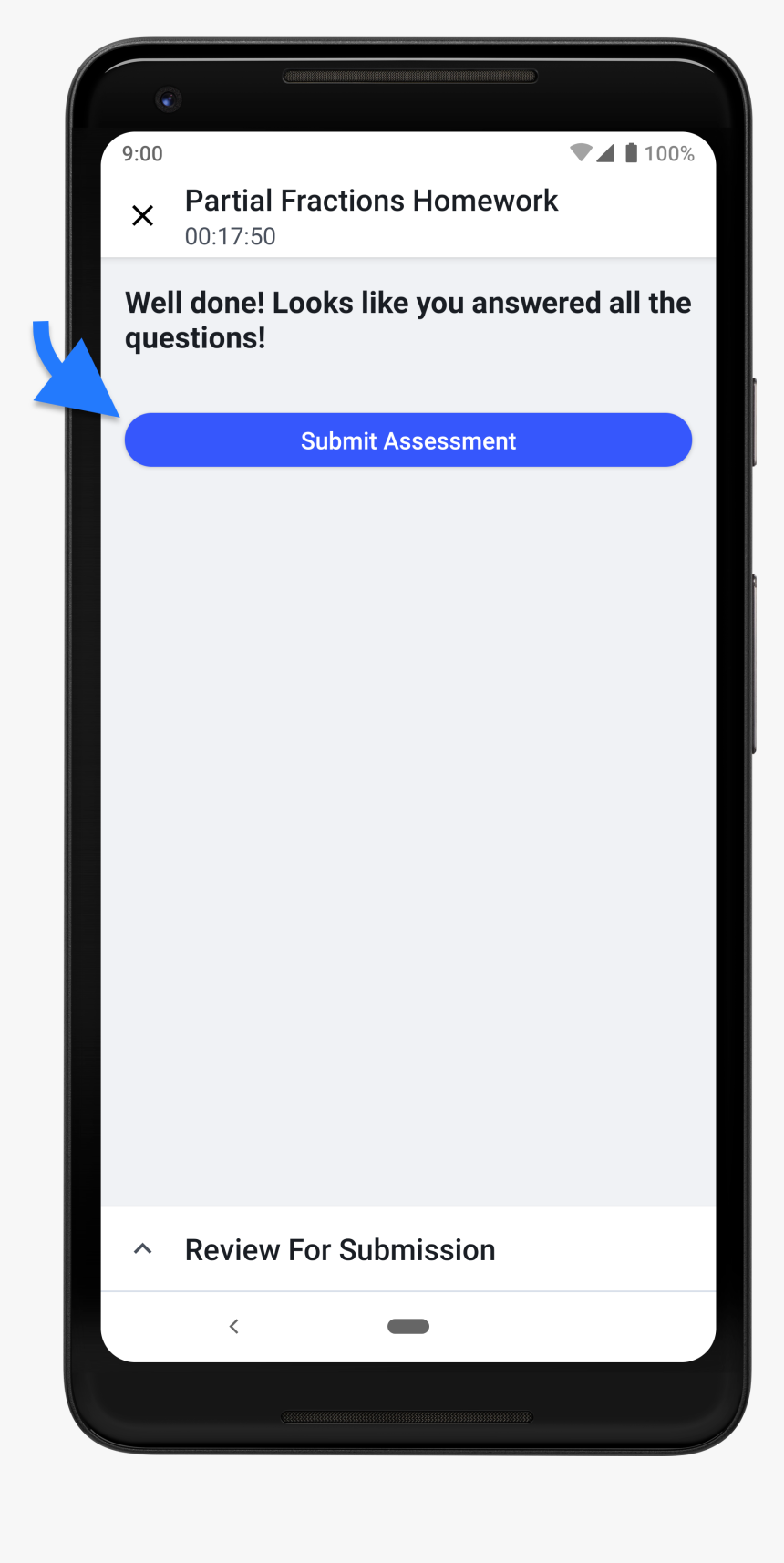The image features a black cell phone prominently displaying a screen with various elements. The phone's side buttons are clearly visible. The top-left corner of the screen shows the number "9," while the top-right corner displays Wi-Fi and cellular signal bars along with a battery life indicator at 100% charge.

Below these indicators is a header that reads "Partial Fractions Homework" followed by a timestamp of "00:17:50." The central part of the screen, while mostly white with a slight gray hue, contains a congratulatory message stating, "Well done! Looks like you answered all the questions." Directly beneath this message is a large blue button with white text labeled "Submit Assessment."

Overlaying the top portion of the phone's screen from the side of the image is a blue arrow pointing directly at the "Submit Assessment" button, suggesting it was added in post-editing. At the very bottom of the screen, text reads "Review for Submission," separated by a prominent dark black line.

Overall, the image is dominated by white space, with the screen's active content occupying a much smaller area. The notable colors in the image are black, white, gray, and blue, with the empty white space comprising roughly three-fourths of the visible screen area.